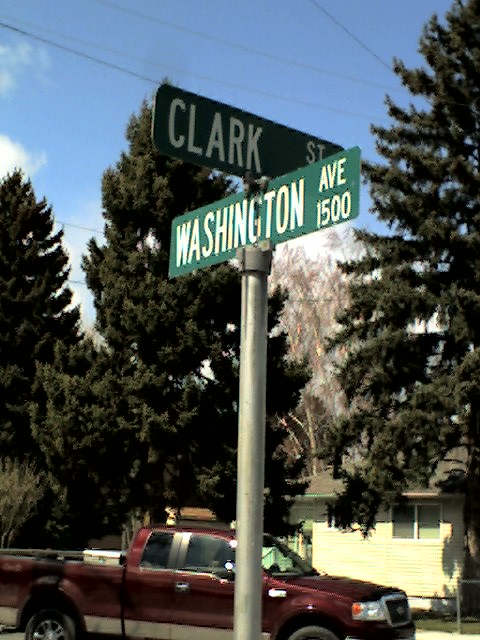This vertical rectangular photograph captures the intersection of Clark Street and Washington Avenue. Central to the image is a tall cylindrical steel pole featuring green street signs with white text. The upper sign reads "CLARK ST" in all caps, while the lower sign indicates "Washington Ave 1500." Sunlight highlights the "Washington" sign, accentuating its details. The picture frames a maroon pickup truck with an open back and a large silver toolbox parked on the street. Behind the truck, a small beige-yellow house, partially obscured by the frame, is enclosed by a cyclone fence and a neatly kept lawn. Towering fir trees, along with a mix of other broadleaf trees, dominate the background, reaching up into a cool blue sky adorned with some clouds and scattered cables. The scene captures a quiet neighborhood intersection on a clear day.